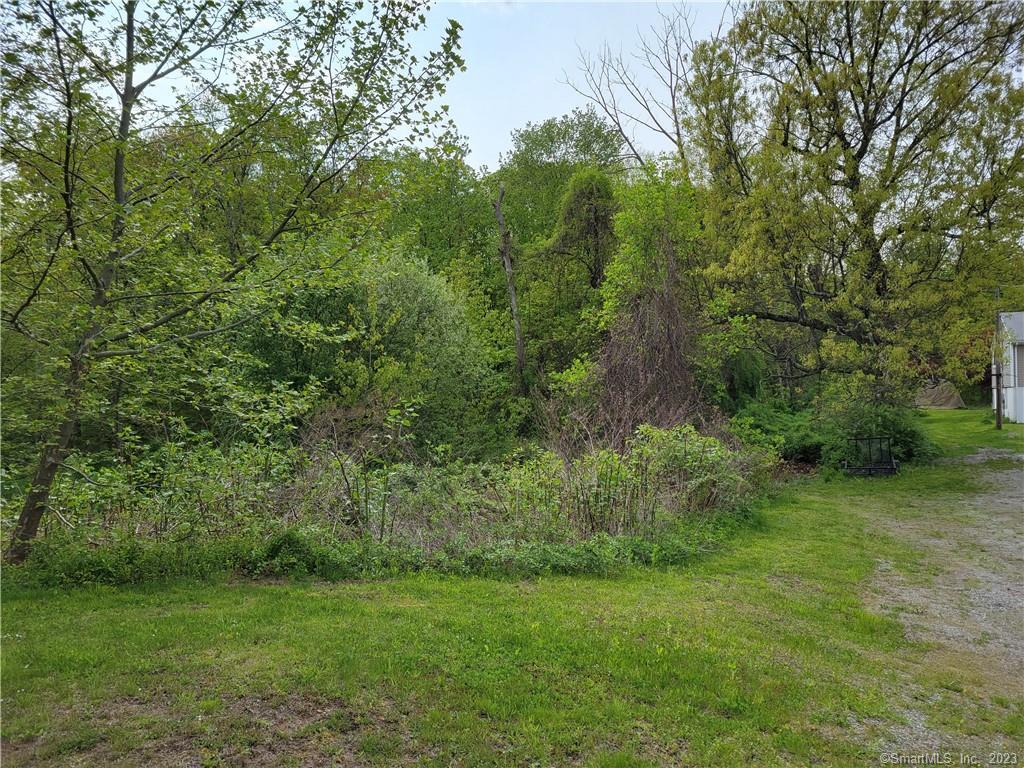This image depicts a tranquil nature scene on a clear, daytime sky adorned with faint clouds. Dominating the foreground is a mixed patch of light and dark green grass, interspersed with a few brown patches. The grassy area extends into what appears to be a wooded boundary, where various green trees stand tall, though some exhibit dead branches and leaves. On the right side of the image, spilling over into the grass, is a spread of gravel hinting at a nearby driveway. A small section of a white building, possibly a garage or part of a house, is visible on the center-right edge of the photograph. The background is filled with the tops of additional trees, adding depth to the serene landscape. The image is slightly branded with white text at the bottom right that reads "SmartMLS Inc. 2023".